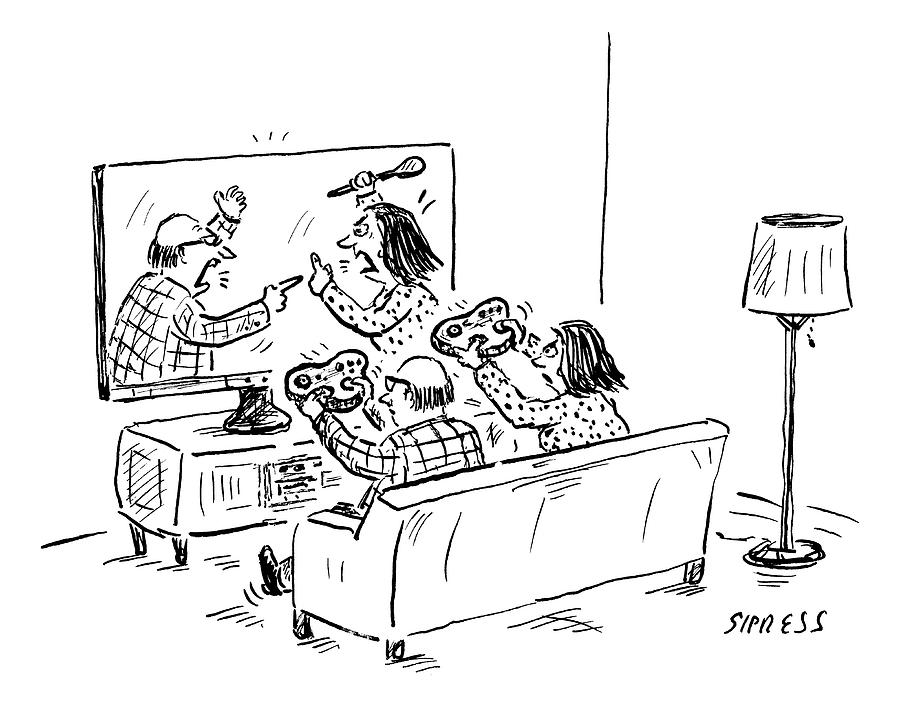The image is a simple black hand-drawn comic sketch, reminiscent of newspaper strips, with a stark white background depicting a living room setting. A man and a woman are seated on a sofa facing a large flat-screen TV, with a long night lamp visible to their side. The man, who is bald and wearing glasses, is holding a giant video game controller with his arms stretched out in front of him. The woman next to him mirrors his actions, also holding a game controller. On the TV screen, both characters are shown in an animated argument: the man is shouting at the woman, while she points a finger at him with one hand and raises a wooden spoon in the other, poised to strike. In the bottom right corner of the image is the artist's signature, "Sipnis."